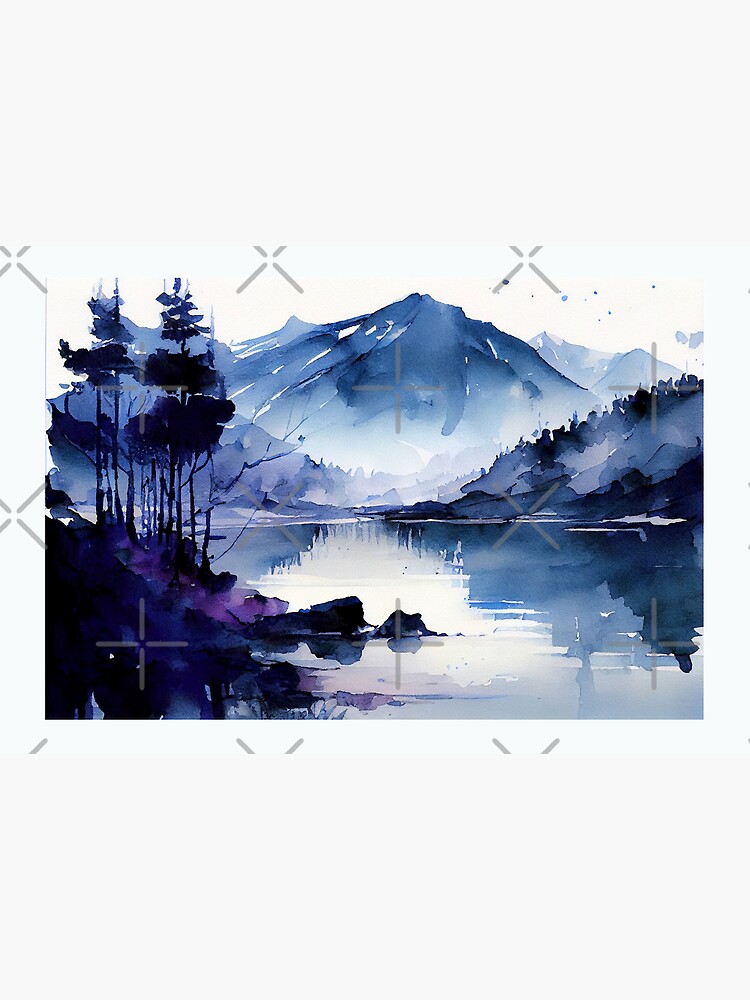This image features a rectangular portrait-style canvas primarily dominated by white space. Nested within is a smaller rectangular landscape artwork that appears to be a watercolor painting. The scene portrays mountains, trees, and a lake with the mountains’ reflections. The colors range from deep blues and purples to light blues fading into white, giving it a tranquil, ethereal quality.

In the foreground, an island extends from the left side, adorned with trees reminiscent of a Bob Ross painting. The distant mountains are the centerpiece, framed by additional background mountains and reflecting partly on the lake. However, the trees near the water reflect more prominently than the mountains themselves.

The image appears to have a watermark overlay, with gray cross marks suggesting it's an unlicensed photo. This composition, abstract in its artistic execution, would be suitable for hanging on a wall, perhaps as a canvas painting available for sale.